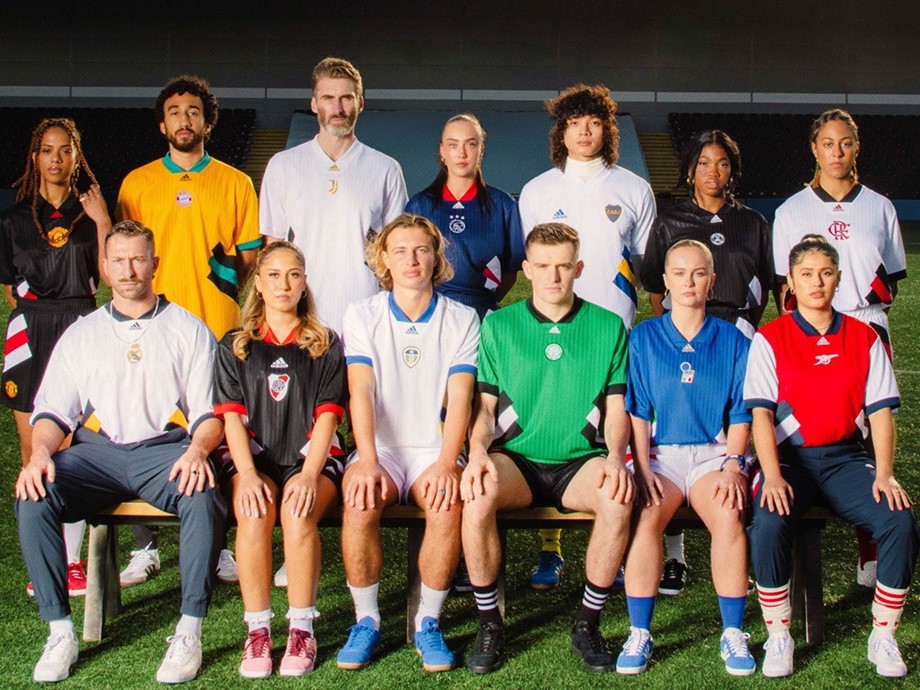This is a detailed photograph taken outdoors, likely inside a stadium, showcasing a diverse group of soccer players seated and standing in front of a set of audience stands with a large concrete wall visible behind them. There is a mix of male and female players, organized with about six players sitting on a bench in the front row and seven players standing behind them. The athletes hail from different teams, wearing a variety of uniforms in red, blue, green, white, black, and yellow, suggesting representation from different nations. The ground beneath them is AstroTurf. Focused attention is drawn to a woman standing on the right side of the image, who is adorned with earrings and dressed in a combination of red, white, and blue shirt, dark blue pants, white shoes, and red and white socks. Next to her is another woman with blonde hair and earrings, wearing a blue shirt, white shorts, and blue socks. The mix of ethnicities among the players further highlights the photograph's diversity.